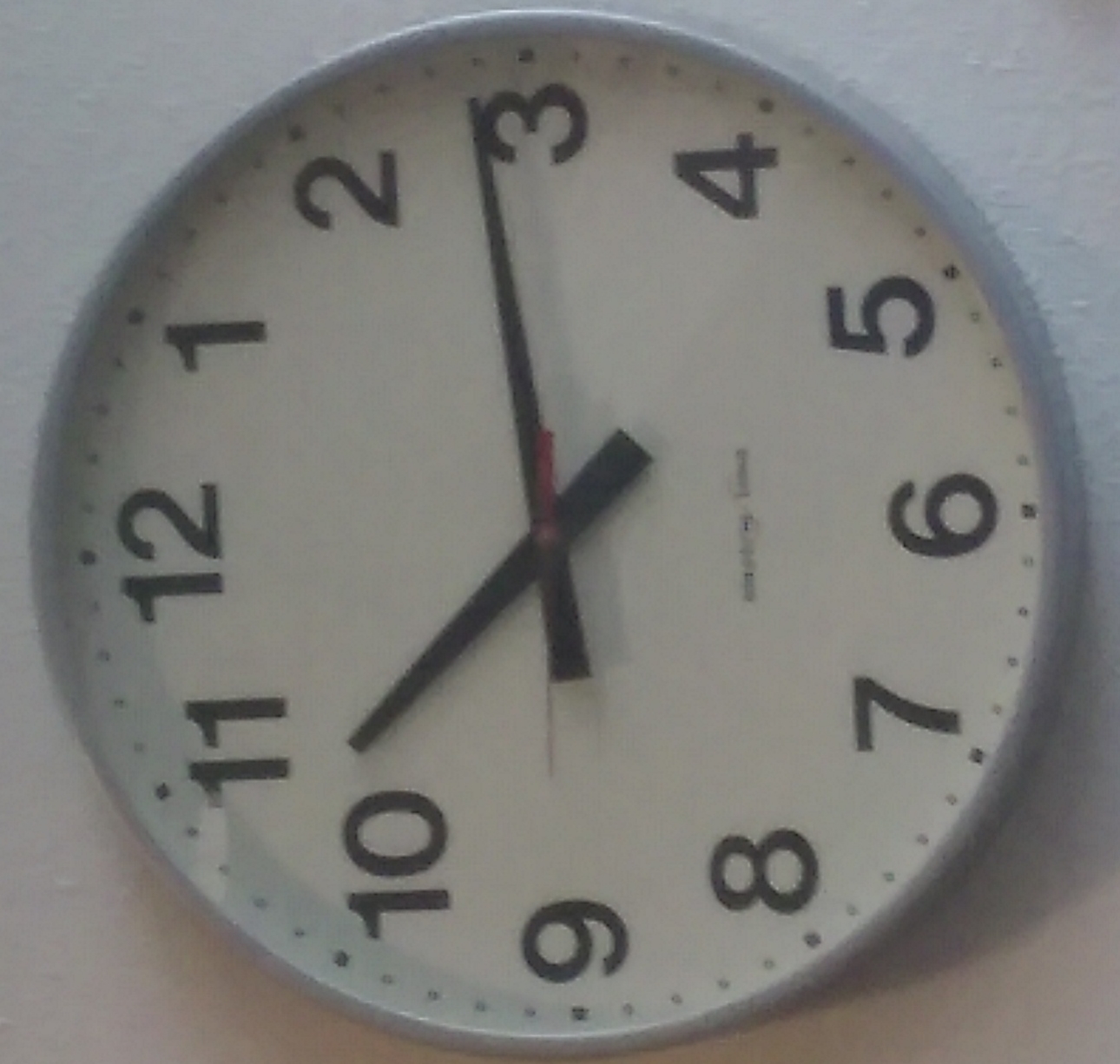This image features a close-up of an analog wall clock. The clock face is primarily white, adorned with sleek black numerals that clearly denote each hour. A striking red second hand contrasts against the black hour and minute hands, all encased in a polished chrome border that adds a touch of modern elegance. The lower half of the clock, just above the number six, has some text, presumably the brand or model name, although it is unreadable due to the image's blurriness. The overall photo quality is quite grainy, and the clock appears to be positioned against a white stucco wall. Notably, the clock (or possibly the entire image) is tilted slightly to the left, suggesting it might have been hung unevenly. The current time displayed is approximately 10:14.